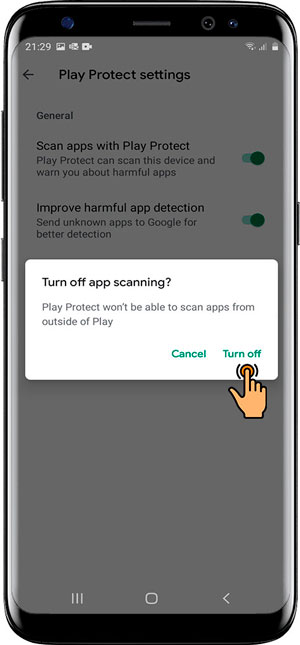The photograph showcases a typical smartphone characterized by black bezels surrounding a central screen. The time displayed at the top of the screen is 21:29. Adjacent to this, on the left, is a gallery icon represented by a white photo symbol. On the right side of the status bar, the device indicates full Wi-Fi and mobile signal strength, with the battery level at 50%.

The primary content of the screen is a gray interface with distinct sections and text in black font. The main heading reads "Play Protect Settings," followed by a subheading titled "General." Under this, an active setting labelled "Scan Apps with Play Protect" is described, which indicates that Play Protect is enabled to scan the device for harmful apps. Another active setting, "Improve Harmful App Detection," follows, suggesting that the device will send unknown apps to Google to enhance app detection.

At the bottom, a white rectangular pop-up menu displays a message in black font that queries, "Turn Off App Scanning? Play Protect won't be able to scan apps from outside of Play." Below this prompt are two options: "Cancel" and "Turn Off." Accompanying the "Turn Off" option is a small icon depicting a human hand poised to click the button.